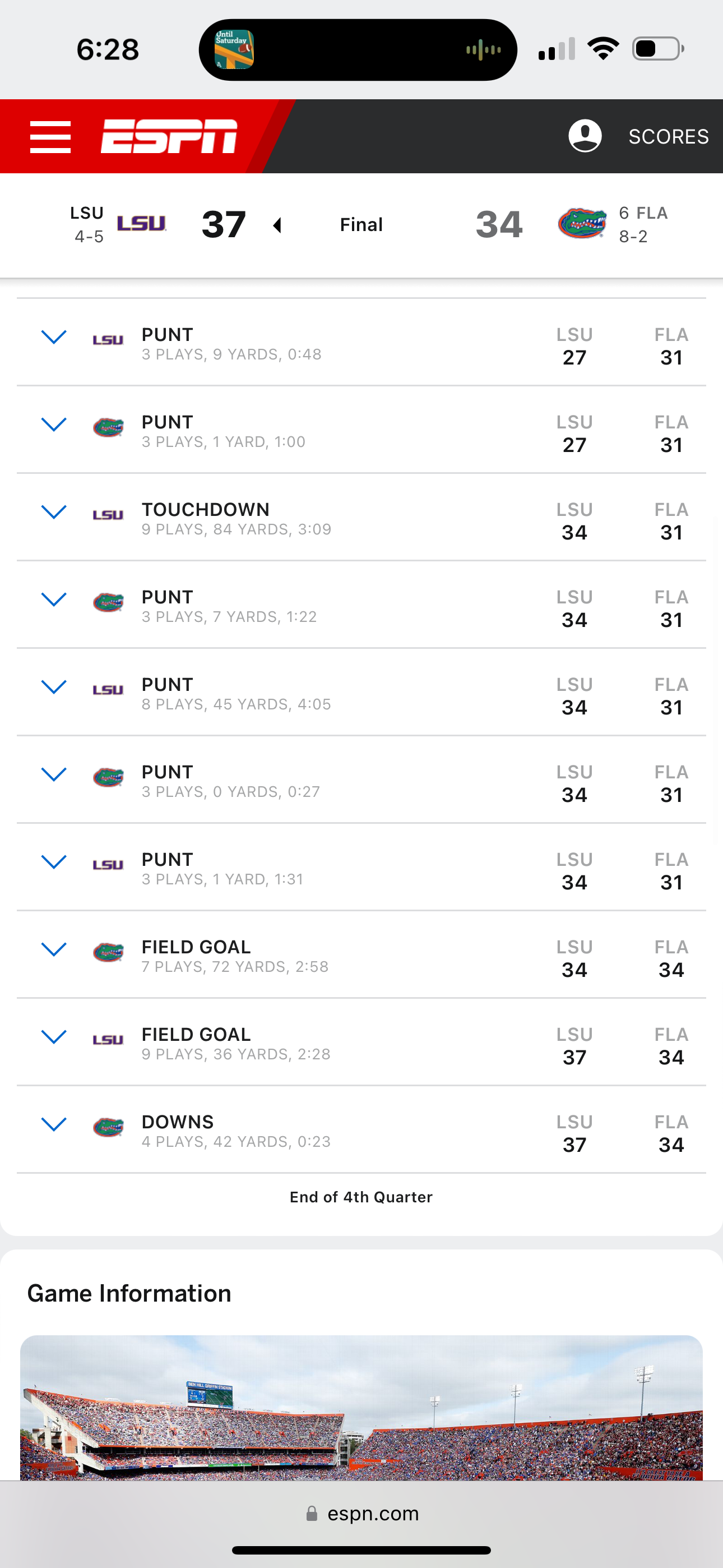The screenshot depicts a mobile device displaying the ESPN app interface. At the upper left corner, a light gray header shows the current time, "6:28," in a black Arial-type font. In the top center, a long black oval houses an icon indicating that a video is playing audio, represented by varying grey lines suggesting an audio stream. On the right side of the header, the device signal strength is shown as "2 out of 4" bars, alongside a black WiFi icon. Further right, a battery icon with approximately half charge is outlined in black.

Beneath the header, there is a vibrant banner with a red background. On the left side of the banner are three horizontal white lines, followed by the ESPN logo in white on the right. The banner culminates in a slant, directed upwards to the upper right with a darker red border, transitioning into a dark gray background.

On the far right of this banner, a white circle contains a dark gray silhouette of a user icon. Adjacent to this, the word "SCORES" appears in uppercase white lettering. Below this banner, another appears with a white background. Towards the left side in small capital letters is "LSU," followed by "4-5" underneath. To the right, in bold digitized grey lettering, the text "LSU" appears once more.